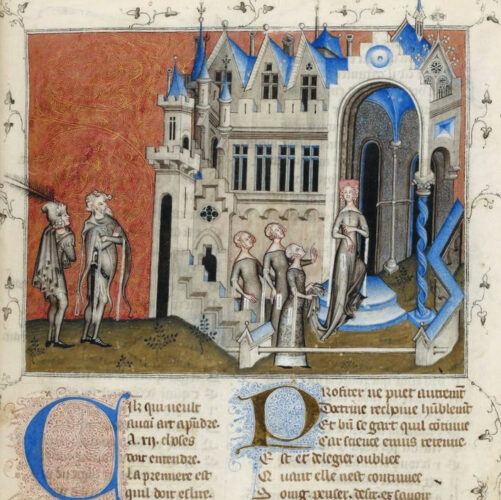The image is a detailed, color illustration reminiscent of a medieval illuminated manuscript, presented in landscape orientation. This shows the upper half of an illustrated page from a manuscript of Guillaume de Machaut's "Le Remède de Fortune," published by the Bibliothèque Nationale in Paris. The scene captures the author arriving at the castle of his lady, rendered in a style that suggests medieval illumination but with some elements that appear more modern, possibly from the Victorian period. The illustration depicts a castle on the right side, with a woman in a medieval gown standing on the steps of the archway. She is accompanied by three female attendants in long gowns. On the left side, two men dressed in court attire, one in a cape-like cloak, are approaching. The background features an orange sky and brown ground, and the entire composition is enclosed by a decorative scroll pattern. Below the illustration, two columns of foreign language text in illuminated manuscript style are visible, featuring ornate initials in blue and brown.